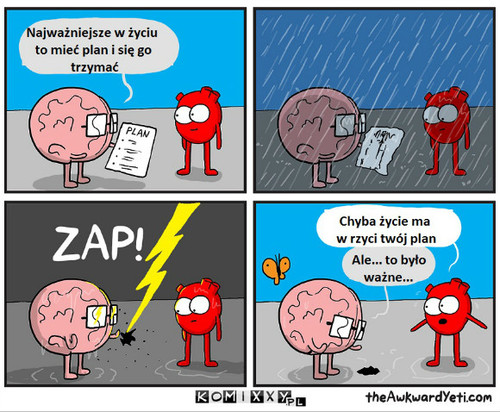The image is a four-panel comic strip by TheAwkwardYeti.com, depicting a humorous interaction between a brain and a heart, with text in an unidentified language. In the first panel (upper left), the brain, characterized by wearing glasses and holding a plan, is explaining it to the heart, which has large white eyes and a concerned expression. Both characters have speech bubbles above them. In the second panel (upper right), it starts to rain, causing the ink on the brain's plan to smudge. By the third panel (lower left), a lightning bolt strikes, dramatically zapping the plan out of the brain's hands and further soaking both characters. The final panel (lower right) shows the brain and heart standing amidst the remnants of the burned plan, with the brain looking sad and the heart still concerned. A butterfly flutters behind them in the now sunny setting, as they exchange words in speech bubbles that remain indecipherable. The comic strip suggests a comedic yet poignant moment of plans going awry due to unforeseen circumstances.